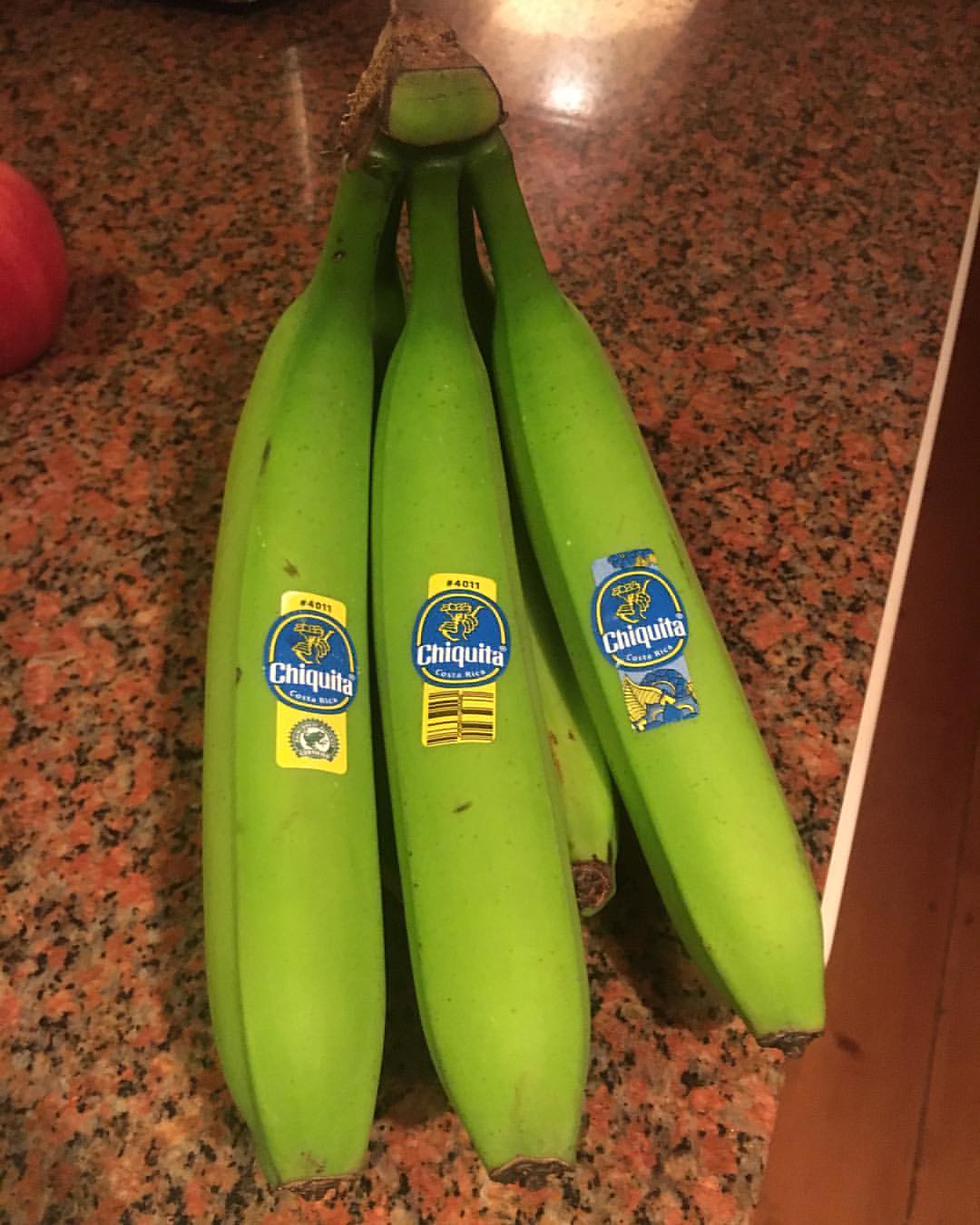The image is a detailed photograph taken indoors, featuring a vertical rectangle shape. The main focus is a central bunch of unripe, green Chiquita bananas, consisting of five bananas connected by their stems at the top. Each visible banana prominently displays a Chiquita sticker, which is yellow with white text inside a blue circle. The arrangement includes three bananas on top with slight variations in the sticker designs, and a fourth banana peeking out from beneath the front bananas.

The bananas rest on a shiny granite countertop or table with a reddish, brown, black, and pink speckled pattern, giving the surface a textured and polished appearance. To the bottom right of the image, part of a medium brown wooden floor is visible. Additionally, in the upper left corner, a small portion of either a red apple or a peach is partially seen, adding a touch of contrast against the speckled granite background. Light reflecting off the countertop enhances the vivid colors and details of the scene.